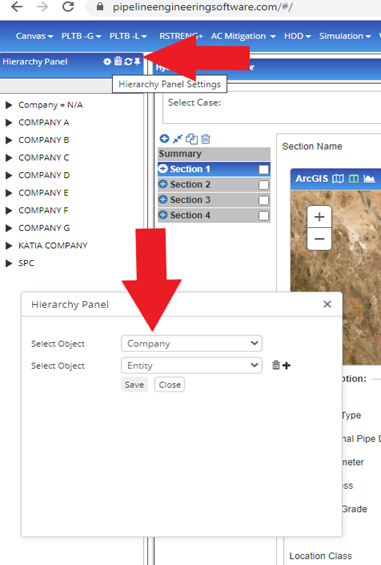This detailed screenshot features a web-based pipeline engineering software interface. Prominently displayed is a hierarchy panel that lists various companies, including Company A, Company B, and Company C. Users can navigate between different companies by expanding this list.

A pop-up window labeled "Hierarchy Panel" is also visible, offering configuration settings for the user. Within this window, two drop-down menus are accessible: one labeled "Select Object" with the company option selected, and another "Select Object" with the entity option selected. Additionally, there are buttons for saving configurations and closing the window.

Another section labeled "Select Case" is present, summarizing multiple sections such as Section One, Section Two, Section Three, and Section Four. The interface also includes a map view accompanied by a toolbar that provides different map functionalities.

A red arrow highlights the hierarchy panel button along with the pop-up window's panel settings configuration. This indicates the software's capability to pin the hierarchy panel, allowing users to select or pin specific companies as needed for their tasks. This tool facilitates efficient navigation and configuration within the software.